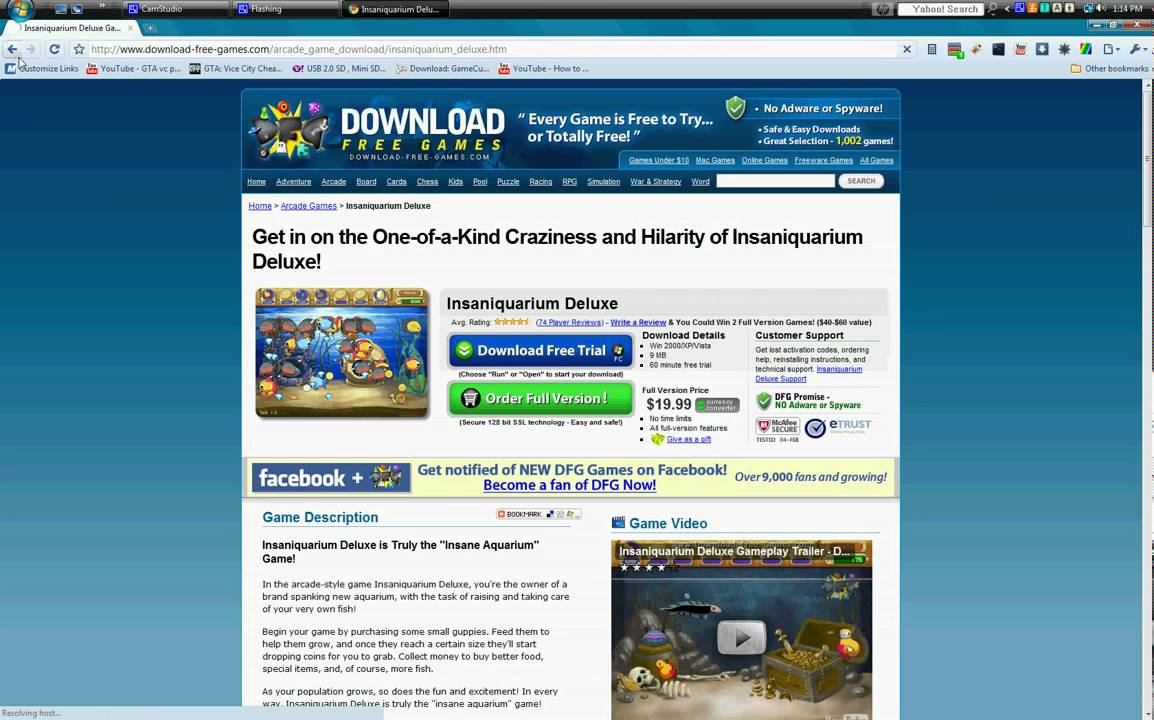Here is a cleaned-up and detailed caption for the image described:

---

**A Vertical Promotional Newsletter Displayed on a Turquoise Gradient Computer Screen**

The image showcases a vertical promotional newsletter displayed on a computer screen with a background gradient of turquoise blue, transitioning from a darker shade at the top to a lighter one at the bottom.

At the top of the newsletter, a blue horizontal banner features the text "DOWNLOAD" in all capital white letters. Directly below, in slightly smaller all-capital yellow letters, it reads "FREE GAMES." To the right of this section, a white quote reads, "Every game is free to try or totally free." Continuing to the upper right corner, another white text states, "No Adware or Spyware," followed by additional unreadable text.

The main body of the newsletter has a white background. At the top, in bold black font, it proclaims, "Get in on the one-of-a-kind craziness and hilarity of Insane Aquarium Deluxe!" Below this statement is a horizontally rectangular image of the game, though the details are hard to discern. To the right of the game image, in bold black font, the title "Insane Aquarium Deluxe" is reiterated.

Beneath this section, two horizontal rectangles are visible. The first is a blue rectangle with the text "DOWNLOAD FREE TRIAL" in all capital white letters. Below it is another rectangle sporting a neon green background with the words "ORDER FULL VERSION," also in white capital letters. To the right of this, the price "$19.99" is displayed in black font.

Further down, a pale yellow horizontal section contains the Facebook logo on the left with the word "facebook" plus the symbol "+" in white lowercase letters within a blue background. Adjacent to this, in blue font, it invites users, "Get notified of NEW DFG games on Facebook!". Centered in a brighter blue section below, it encourages, "Become a fan of DFG now!". To the right, it proudly announces in blue font, "Over 9,000 fans and growing."

At the bottom of the newsletter, the words "GAME DESCRIPTION" are written in turquoise or teal lettering. Following this, a bolded black text reads: "Insane Aquarium Deluxe is truly the 'Insane Aquarium' game!" An article in smaller black text follows this description, providing further details. To the right, another scene from the game, depicting an underwater environment, is visible.

---

This caption provides a comprehensive and detailed description of the promotional newsletter, covering all visible elements and their specific locations within the image.